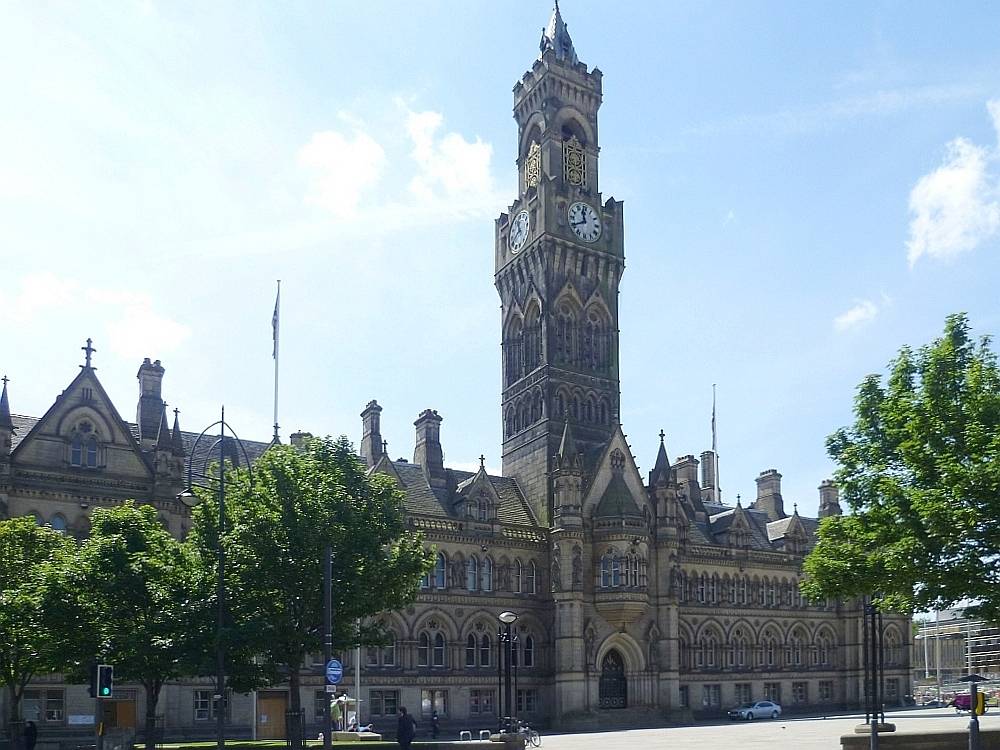This photograph, taken outdoors during the daytime, captures a grand, multi-storied building steeped in old architectural style, reminiscent of the Victorian era. Central to the image is a towering clock tower, rising significantly above the four-story building and featuring traditional clock faces on its visible sides. Adorning the rooftops are multiple church crosses, underscoring the building's ecclesiastical nature. In the foreground, a courtyard is visible with one person walking and a white car parked nearby. Trees frame the scene, positioned at the front left and back right, adding a touch of nature to the urban setting. The sky is a bright blue with some wispy white clouds, whiter towards the left where the sun shines intensely. The paved ground below the building extends into a walkway or courtyard, and in the distance on the right, smaller buildings and street lamps can be seen, enhancing the cityscape ambiance.